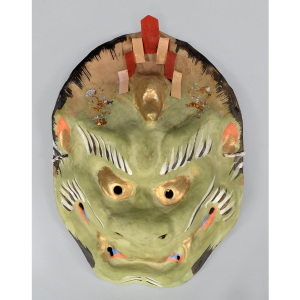This close-up photograph captures a ceramic mask that resembles a dragon and exhibits features suggestive of Mayan artistry. The mask is mounted on a semicircular wooden board, which mirrors the width of the dragon's head and is decorated with black streaks around its edges. The dragon's complexion is a pale, gray-green, adorned with large, golden eyes speckled with black pupils. Its eyebrows are artfully depicted through black and white brush strokes, extending similarly over the cheekbones, adding a striking contrast.

The dragon mask exhibits human-like features such as a broad nose, set off by meticulously painted whiskers stretching from the corners of its grinning mouth back towards its small, pink ears, which are subtly dotted with gold on the inside. The inner corners of its mouth feature vibrant pink and blue streaks for added detail. 

Atop its head, the mask wears an ornamental hat, styled in an oriental Maya theme, comprising a black half-circle with tan hues below and dripping black accents. Attached to this hat is an intricate arrangement of red, cream, pink, and gold rectangular pieces of construction paper, the latter matching the dragon's eyes and forming a prominent centerpiece. All these elements are set against a contrasting lilac background, emphasizing the mask's rich detail and diverse textures.